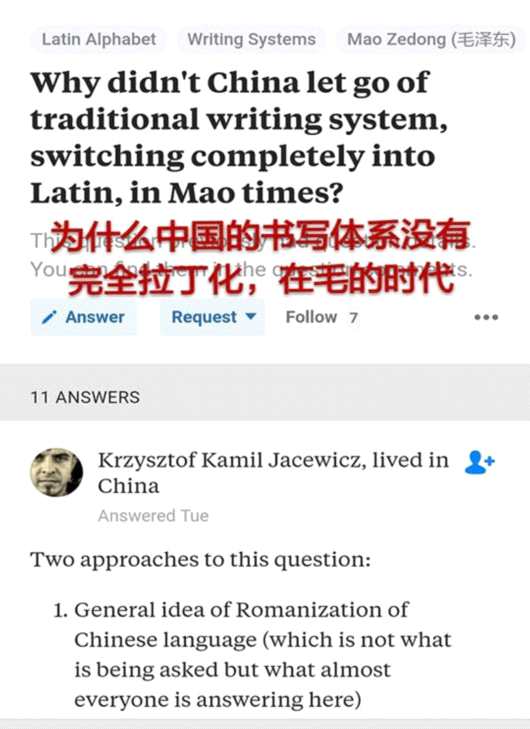The screenshot depicts an article discussing why China refrained from fully adopting the Latin alphabet during Mao's era, opting to maintain traditional Chinese writing systems instead. The article’s title is visible, along with several Chinese characters overlaying it. Below the title, there are details indicating that the post has 711 answers and includes requests for additional responses and followers. The content visible in the screenshot highlights two central approaches to the question: the first approach discusses the general notion of the Romanization of the Chinese language, which appears to be the focus of many responses, although it is not directly addressing the core query. The rest of the answer is truncated, and the name of the person providing the answer is not readable.